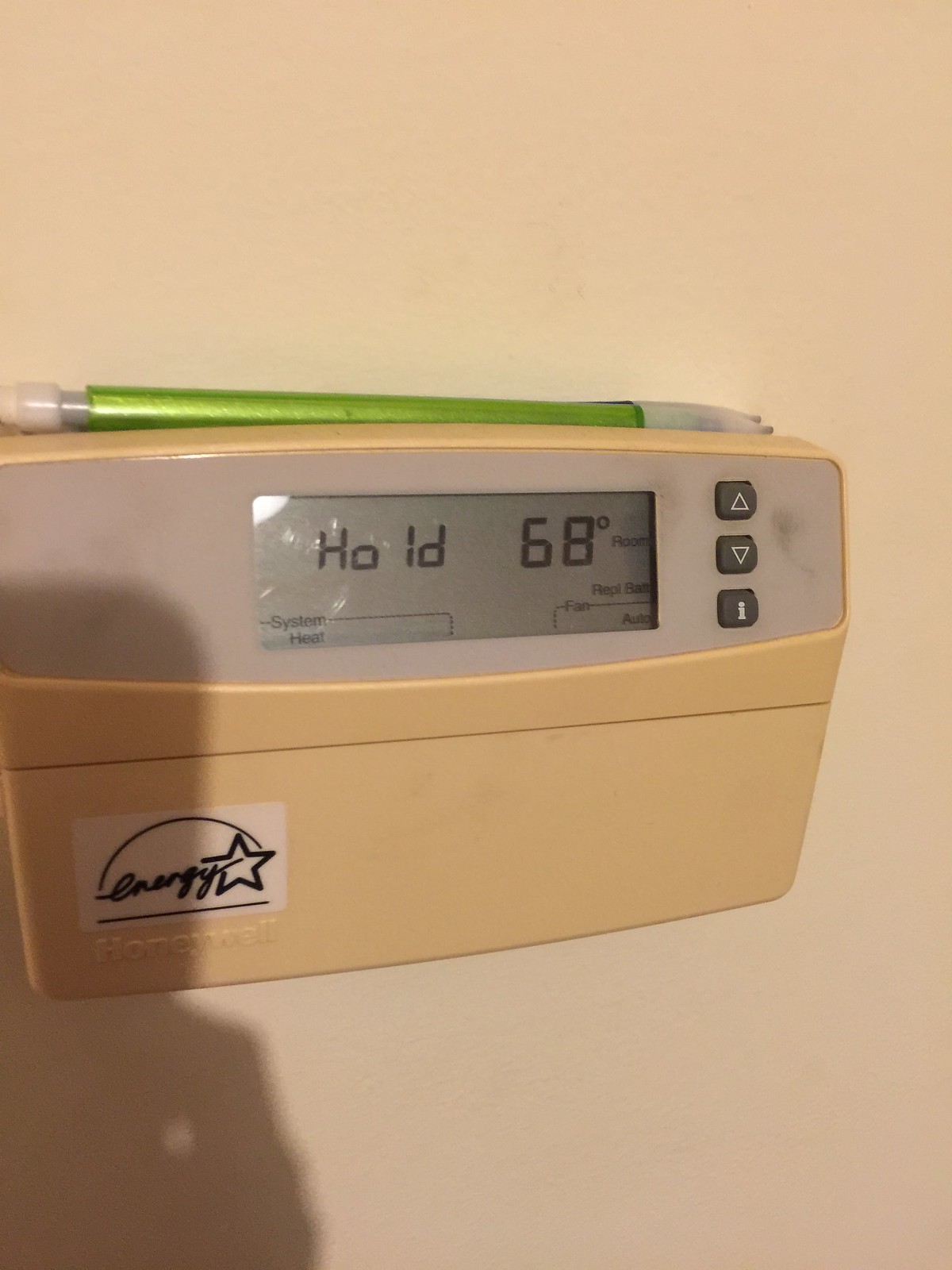This detailed indoor photograph, taken at a slight angle to a white wall, features a rectangular digital thermostat as the centerpiece. The thermostat, prominently positioned on the wall, displays an LED screen in its upper half. The screen has dark digital letters that display the word "hold" to the left and the temperature "68°" to the right. Adjacent to the display, on the right side, there are three vertically arranged buttons: the top button with an upward-pointing white triangle, the middle button with a downward-pointing white triangle, and the bottom button with a small lowercase "i."

The thermostat case is light tan, almost dirty in appearance, particularly noticeable at its lower section. In the lower left corner of the thermostat, there is a white triangle containing the word "energy" in script, accompanied by a star to its right. Below this triangle, the word "Honeywell" is embossed in raised white letters on the plastic surface.

Resting horizontally on top of the thermostat is a green mechanical pencil, with its eraser on the left and the tip pointing towards the right. The composition also captures a shadow in the lower right region, revealing the distinct shape of a rectangular cell phone and a finger holding it, indicating that this image was taken with a smartphone.